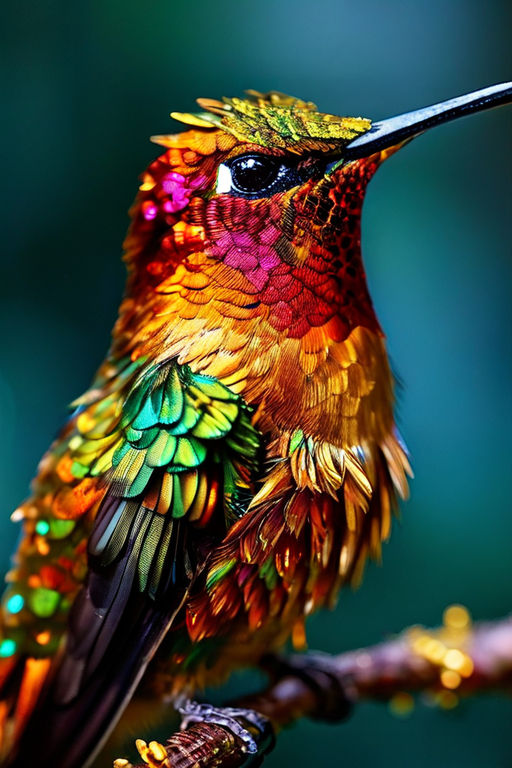This highly detailed image showcases a vibrantly colorful bird resting on a brown branch against a dark bluish-green background. The bird, which appears to be computer-generated or illustrated, is depicted in a side view facing right. It features an array of bright, metallic hues with a distinct, almost unnatural shine. The very top of its head is adorned with vibrant green feathers, transitioning to yellow and orange, while pink feathers surround its black eye. Its long, pitch-black beak is complemented by red feathers below it. The bird's throat is a striking reddish hue that morphs into an orange gradient extending down its neck and stomach. Its wings exhibit a mesmerizing blend of colors, starting with bright green and yellow at the upper section, shifting to blue, and finally to darker black and gray shades towards the tips. Its solid black claws, also shiny and metallic, grip the branch, with the front claw appearing clearer than the slightly blurry back one, adding depth to the composition.